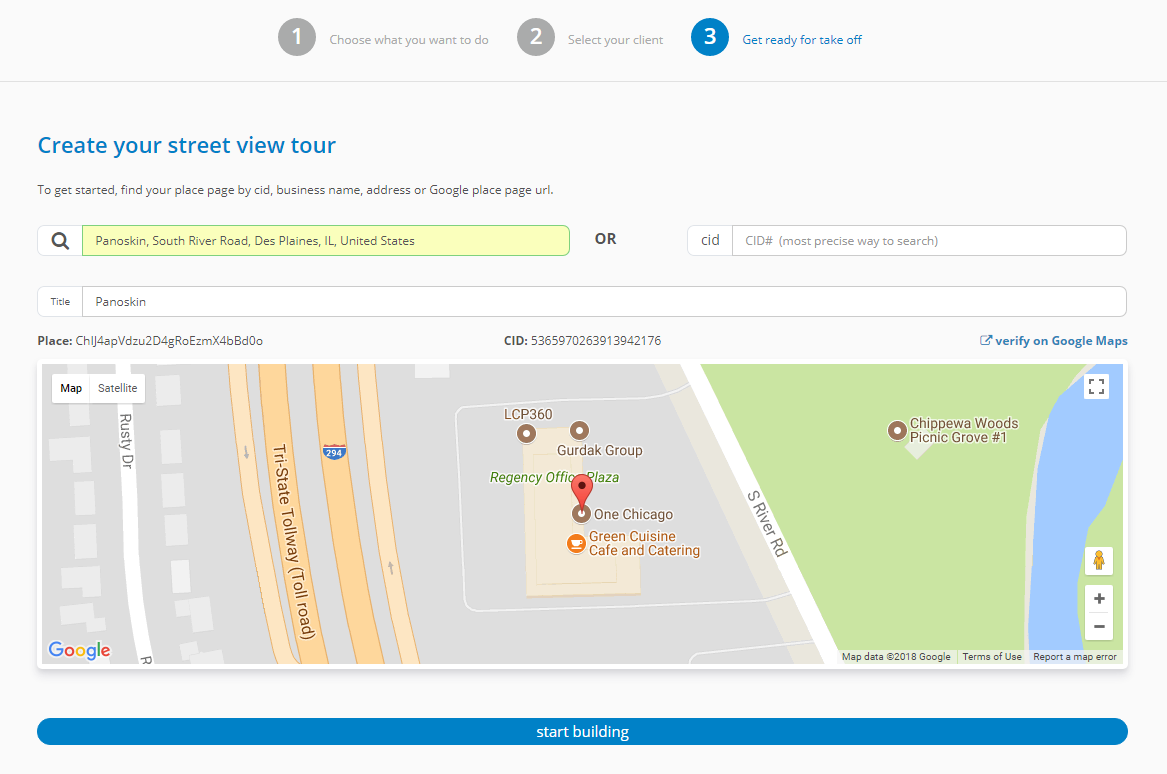Screenshot of Panoskin’s Map Interface for Creating a Street View Tour

At the top, there are three steps listed as options:
1. Choose what you want to do
2. Select your client
3. Get ready for takeoff

At the bottom, instructions read:
“Create your Street View tour. To get started, find your place page by CID, business name, address, or Google place page URL.”

Below this description, a search bar populated with "Panoskin South River Road, Des Plaines, IL, United States" is shown. Adjacent to this is another search bar labeled for the CID input, which is currently empty.

Central to the interface is a detailed map featuring various locations, prominently displaying a pinned location labeled "Chicago Green Cuisine Cafe and Catering." The map has a blue background with identifiable roads and landmarks around it. To the right, a road marked “Tri-State Tollway (Toll Road)” is visible. On the left, a spot labeled “Chippewa Woods Picnic Groove #1” is indicated.

Other notable locations on the map include:
- S River Road
- Regency Office Plaza
- Go-Kodak Groove
- LCP 360

The overall layout of the map interface is designed to assist users in creating and customizing a Street View tour.